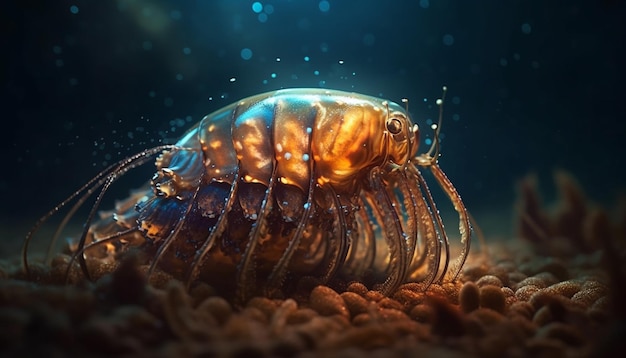The photograph depicts an underwater scene featuring a unique sea creature that resembles a cross between a shrimp, a crustacean, and an insect. The creature, possibly an artistic rendition, has a shiny bronze or golden segmented body with a tiered shell on top. It sports numerous translucent, curved legs—at least ten, with five on each side—moving from the left to the right side of the image. Its body is relatively short, akin to a centipede, but doesn't match the length. Notably, it has two large eyes and antennae extending from the front of its face, and a feathered, brownish tail. The ocean floor, resembling tiny pebbles or beans, adds texture to the setting, which is deeply submerged, as indicated by the dark blue and green hues of the water. Light appears to be filtering down from the top, illuminating the creature against the dark, mysterious backdrop of the sea.